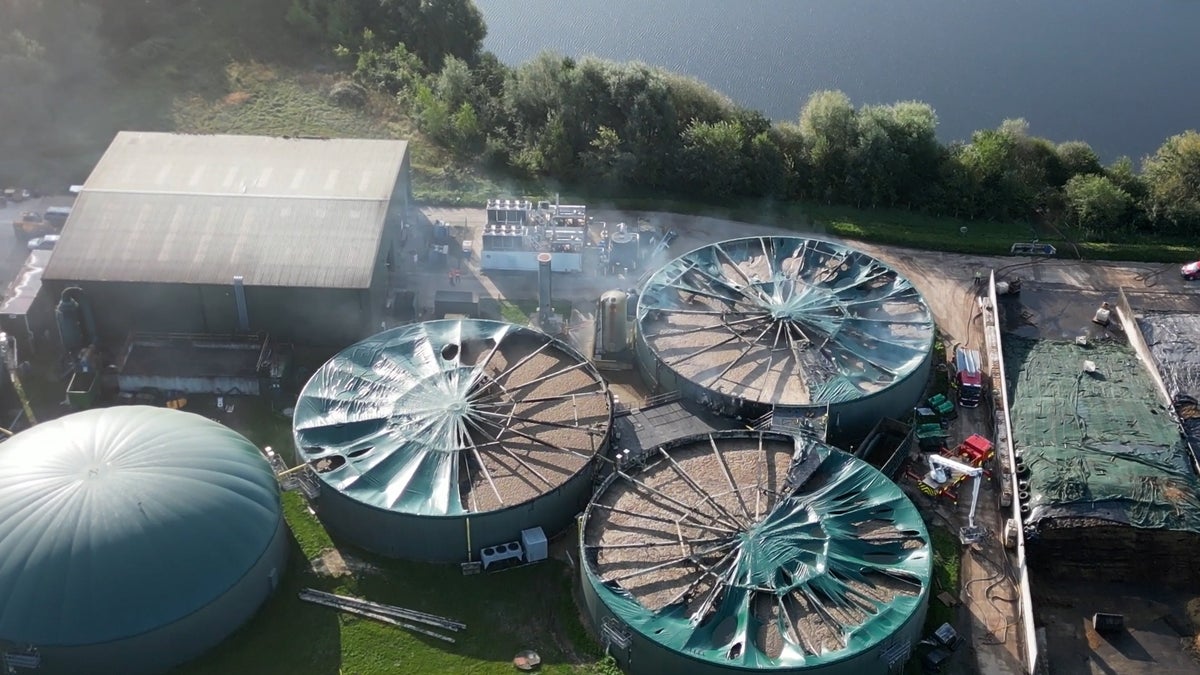This aerial drone photograph captures a large industrial facility that appears to be a wastewater treatment plant or storage facility. At the center of the image, three prominent circular structures are visible, resembling enormous spoked wheels similar to bicycle wheels. These structures are mostly uncovered, with only fragments of green plastic sheeting clinging to the metal spoke frames, exposing the brown material inside, which could be sewage or processed sludge. Adjacent to these, on the left, is a similar green-domed cylindrical tank.

In the upper left corner of the image, a large, rectangular, warehouse-like building features a silver-colored roof. To the right of this building, various industrial equipment is visible, including a cylindrical silver tank, a smokestack, and a crane amid clusters of trucks and construction machinery. This area is enclosed by a wall, beyond which lies a dirt roadway.

In the background, towards the upper section of the photograph, a dense belt of trees and greenery provides a natural boundary, beyond which a blue body of water is visible, adding contrast to the industrial foreground.

Overall, the photograph depicts a juxtaposition of industrial complexity and the natural environment, detailed with dilapidated structures, equipment, and natural elements.